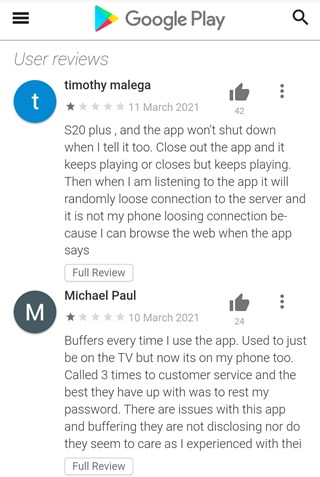In the image, at the very top, there's text in black that reads "Google Play." To the left of this is an arrow pointing right and colored in shades of blue, pink, and yellow, with the text "Google Play" next to it. Below this text, in gray, are the words "User Reviews."

The first review is by a user named Timothy Malega, whose name appears next to a lowercase "t" within a blue circle. Timothy gave the app a rating of 1 out of 5 stars on March 11, 2021. There is also a gray thumbs-up icon underneath the review with the number 42 beside it. Timothy comments, "I spent over $20 on this app, and it won't shut down when I tell it to close. It either keeps playing or closes but continues playing. When I'm listening to the app, it will randomly lose connection to the server. It's not my phone losing connection, as I can still browse the web when this happens."

Below this, another review features a user named Michael Paul, indicated by a letter "M" inside a dark green circle. Michael similarly gave the app 1 out of 5 stars. His review states, "The app buffers every time I use it. Initially, this issue was only on the TV, but now it happens on my phone too. I called customer service three times, and their best solution was to reset my password."